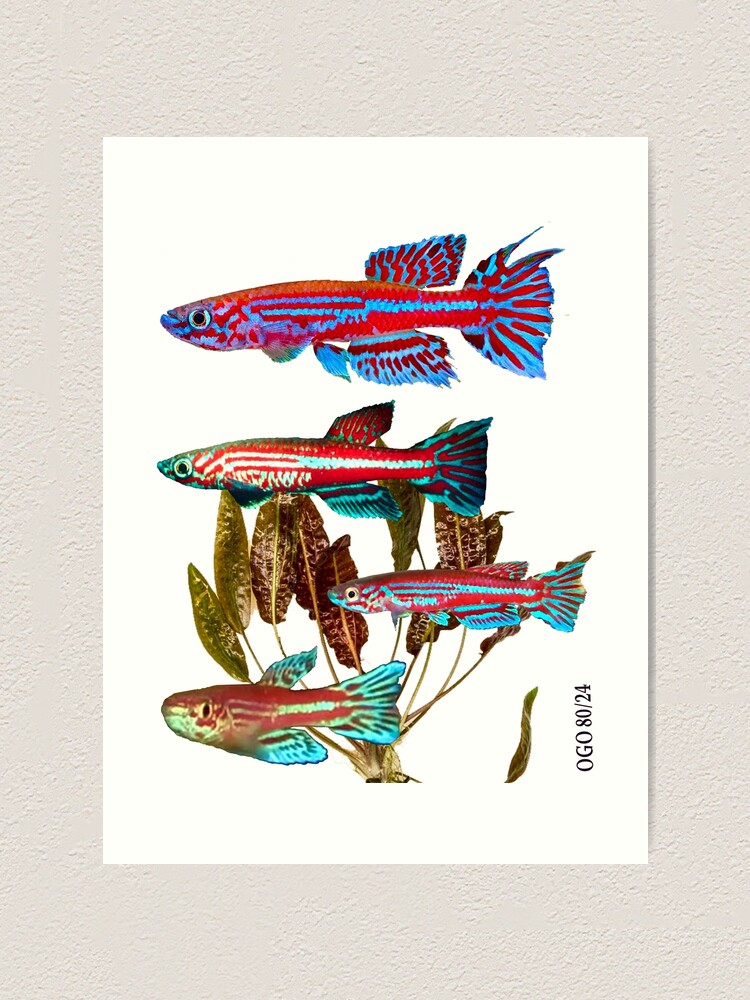This is a detailed photograph of an artistic print hanging on a slightly off-white plaster wall. The print itself is on a piece of distinctly whiter paper and features four vividly colored, long, and skinny guppies. All the fish are oriented with their heads to the left.

At the top of the image is a strikingly long and slender fish with a red body accented by light blue stripes. It has a solid, fan-shaped tail fanned straight behind it, a blue mouth, and a lone visible eye on the side facing the viewer.

The second fish in the middle has a varied and vibrant color scheme: predominantly red and white with a hint of pink. It boasts a turquoise blue tail and bottom fin, a rust-brown or coral-colored top fin, and a distinctive blue snout.

Below this is another fish that closely resembles the top one with a similarly long and skinny build. Its body is reddish-pink with blue lines, mirroring the fanned-out blue tail and blue mouth of the top fish.

The final fish at the bottom stands out with its relatively stouter build. It has two blue fins, a fanned-out blue tail, and a body that is mostly salmon-pink with a yellow highlight along its side, and some white under its nose.

Adding to the composition, a sprig of beige and golden aquatic plants fills some of the white background near the lower fish. On the right-hand side of the print, the text "OGO80-24" is inscribed in black font. The collective visual presentation suggests an artistic intent more than a mere photograph, potentially hinting at a photoshopped creation.